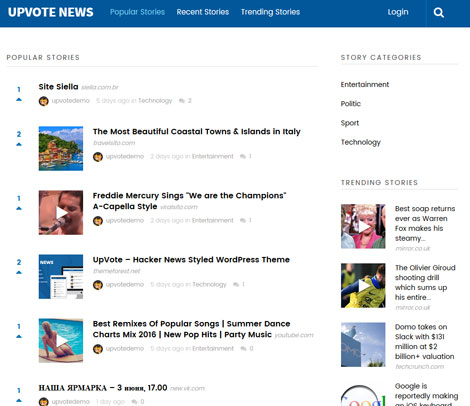The screenshot captures a page from the Upvote News website or app. The interface features a blue horizontal bar at the top with "Upvote News" prominently displayed in bold white text in the left-hand corner. Adjacent to the logo are navigation options for "Popular Stories," "Recent Stories," and "Trending Stories," followed by a login button and a search icon on the right.

The "Popular Stories" section is selected, revealing a list of popular articles against a white background. The stories are as follows:

1. **Cite Stella**
2. **The Most Beautiful Coastal Towns and Islands in Italy**
3. **Freddie Mercury Sings We Are the Champions Acapella Style**
4. **Upvote Hacker News Styled WordPress Theme**
5. **Best Remixes of Popular Songs, Summer Dance Charts Mix 2016**
6. **[Title in Russian Alphabet]**

On the right side, a sidebar presents different story categories, including Entertainment, Politics, Sport, and Technology. Below this, a snippet of trending stories is displayed:

1. **Best Soap Returns Ever as Warren Fox Makes a Steamy…**
2. **The Olivier Giroud Shooting Drill Which Sums Up His Entire…**
3. **Domo Takes on Slack with $131 Million at $2 Billion Plus Valuation**
4. **Google’s Reportedly Making an iOS Keyboard…**

The image primarily showcases the layout and content hierarchy of the Upvote News platform, offering a snapshot of its most engaging stories and user navigation elements.